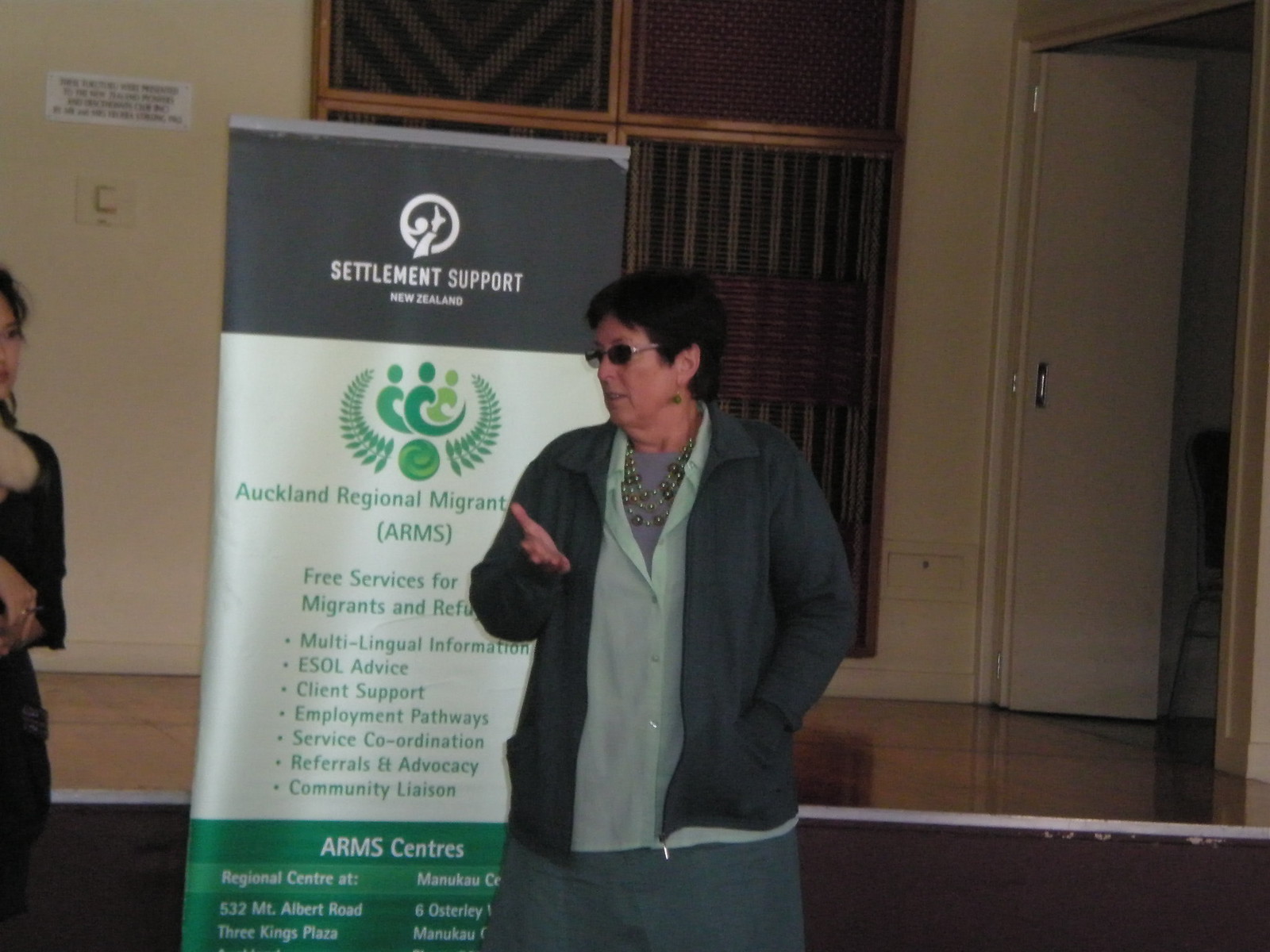In this wide rectangular photograph, a light-skinned woman with dark, short hair is standing in front of a tall rectangular sign that reads "Settlement Support New Zealand Auckland Regional Migrant Arms" in a gray block on the top, with additional information underneath, including "Free Services for Migrants and Refugees," "Multilingual Information," "ESOL Advice," and "Client Support." She is positioned in front of a glossy wooden stage, which has several framed artworks with dark green and reddish colors hanging behind it. To the right of the image is a beige door, while to the left, there is a partial view of a young woman with dark hair wearing a black dress. The main woman is wearing dark sunglasses, a light green transparent blouse over a gray top, and a dark gray skirt or loose pants. She is accessorized with a fancy multi-layered necklace, green earrings, and is holding her right hand palm-up across her shoulder area while her left hand is tucked into her gray jacket.